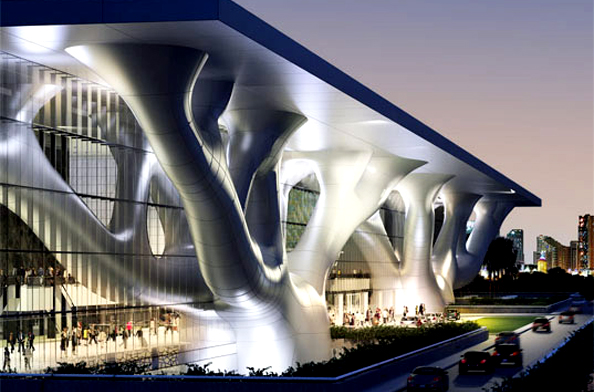This horizontally aligned rectangular image captures an early evening scene featuring a large, modern building with a unique architectural design. The building, which has five stories, prominently displays a striking element—a pair of large, decorative white structures resembling tree trunks or branches, supporting a flat roof with a dark blue border. These tree-like columns are situated towards the left and the center of the image, creating a cutting-edge aesthetic. The building itself is largely composed of reflective glass windows, allowing glimpses of the people inside on the ground level, where a white floor is visible. In front of the building, a narrow gray street runs diagonally from the lower left to the upper right, occupied by cars with their red tail lights on, indicating motion or parking. The sky above is a gradient from light gray at the horizon to a darker gray, symbolizing the transition from day to night. In the distance, particularly on the right side of the image, older and taller city buildings can be seen, providing a contrasting backdrop that emphasizes the modernity of the main building. The scene is accentuated by bands of plants beneath the overhang, adding a touch of greenery to the urban setting.